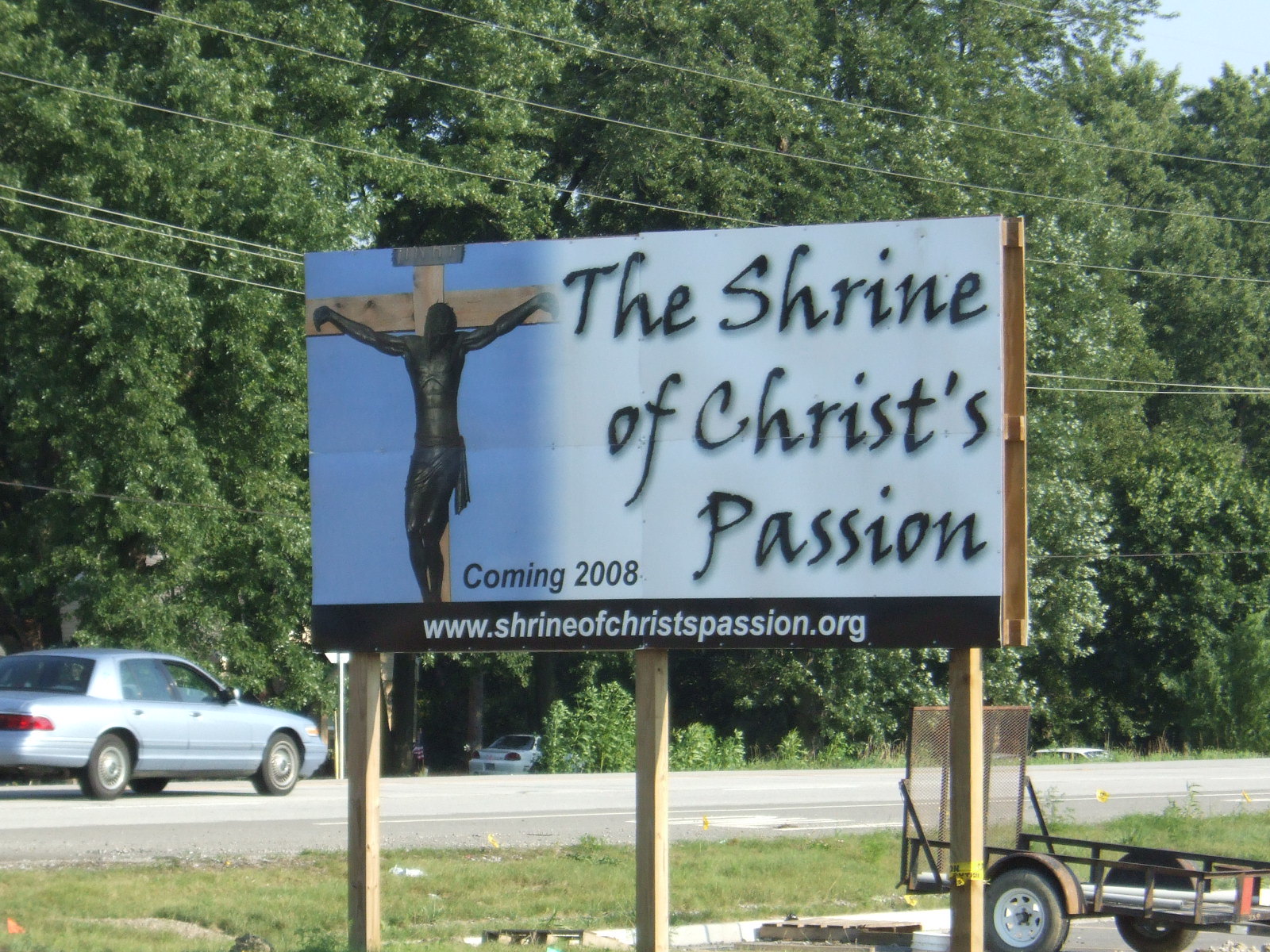The outdoor photograph, taken in landscape orientation, showcases a wooden advertisement near a rural roadway. This short wooden billboard is supported by three pine-colored fence posts. The advertisement features a blue background. The right side of the board displays black, handwriting-style text reading "The Shrine of Christ's Passion". On the left side of the board is a wooden cross, with a cast, black crucifix of Jesus Christ affixed to it. Below the crucifix, in a different black text, the words "Coming 2008" are visible. The bottom strip of the billboard contains a black horizontal banner with white text stating "www.shrineofchristspassion.org". 

The advertisement is positioned adjacent to a light grey asphalt road, which extends diagonally from the bottom left to the back of the image. A blue sedan, resembling a Buick, is visible at the edge of the frame, driving away from the observer. To the right of the billboard, slightly obscured by one of the vertical posts, there is a hitching trailer, likely parked in a nearby lot marked by white curbstones and bordered by a grass verge. In the background, tall, densely-leaved deciduous trees provide a verdant backdrop to the scene, contributing to the rural ambiance. All these elements suggest a North American, rather than British, landscape.